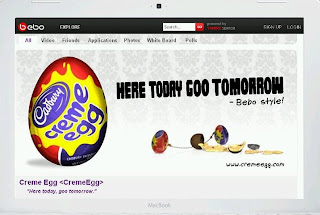The image prominently features a "Creme Egg," spelled as "C-R-E-M-E," indicating non-American English spelling, likely British. The branding on the egg reads "Carbury," and the packaging is primarily purple, while the egg itself is attractively colored in yellow and red hues. The tagline "Here today, goo tomorrow" is displayed, suggesting the egg is partly cracked open to reveal a gooey filling, hinting at its edible, confectionery nature. The company name, "Bibo," is also evident, with distinctive red coloring on the first 'B.'

In addition to the product, the image includes navigational elements from an interface, featuring tabs such as "Video," "Friends," "Applications," "Photos," "Whiteboard," and "Pudis." A search bar is positioned to the right, with the search icon highlighted in red. The top right corner of the interface provides "Sign Up" and "Log In" options. Overall, the captivating visual elements and interface suggest an online platform promoting or selling this intriguing and colorful "Creme Egg."